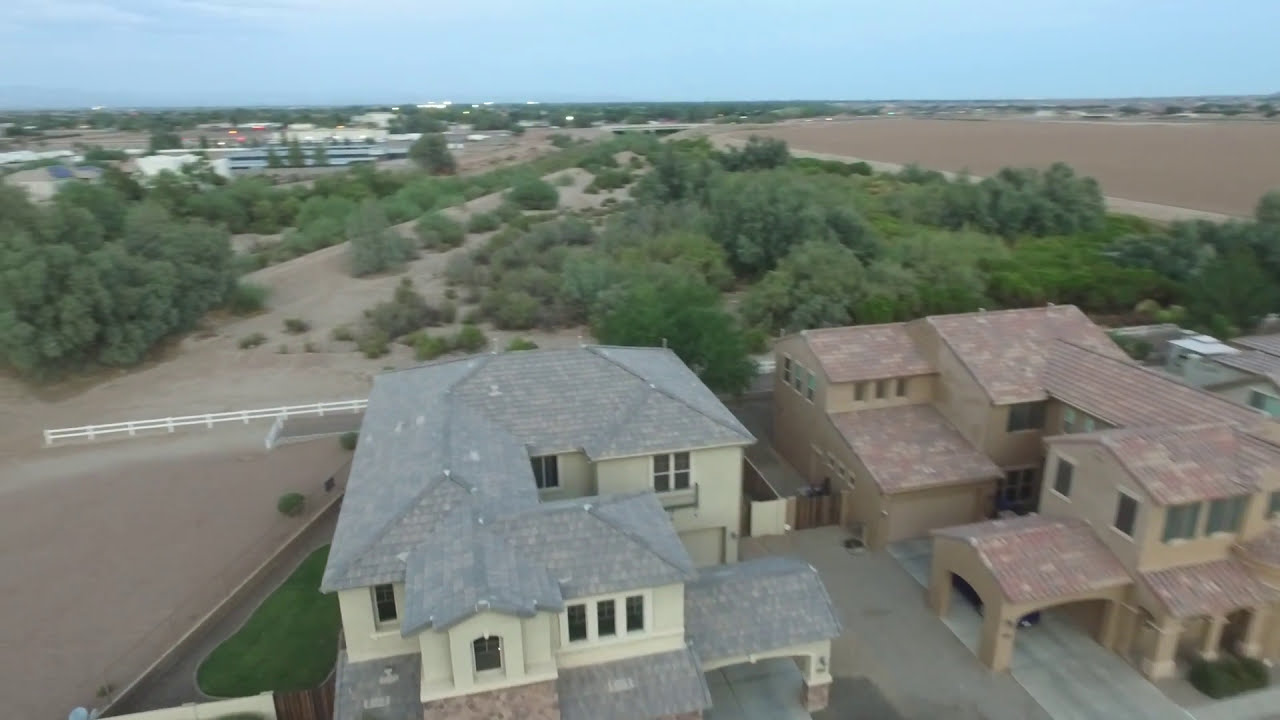This aerial image captures two large, stately homes in a neighborhood foreground, featuring striking similarities in makeup and design. Each home has a spacious, multi-car garage and sits beneath a tile roof—one gray and one brownish-red. The house on the left, painted a lime green or off-white, contrasts visually with its neighbor on the right, which is adorned in a beige or tan color. Both homes appear to cover a sizable footprint, possibly between 5,000 to 10,000 square feet.

The surrounding landscape appears arid, with patches of dirt and sand interspersed with planted trees. In the distance, beyond the immediate neighborhood, lies a field and various places of business, along with additional residences. The sky overhead is a deep, vivid blue, adding a serene backdrop to the scene.